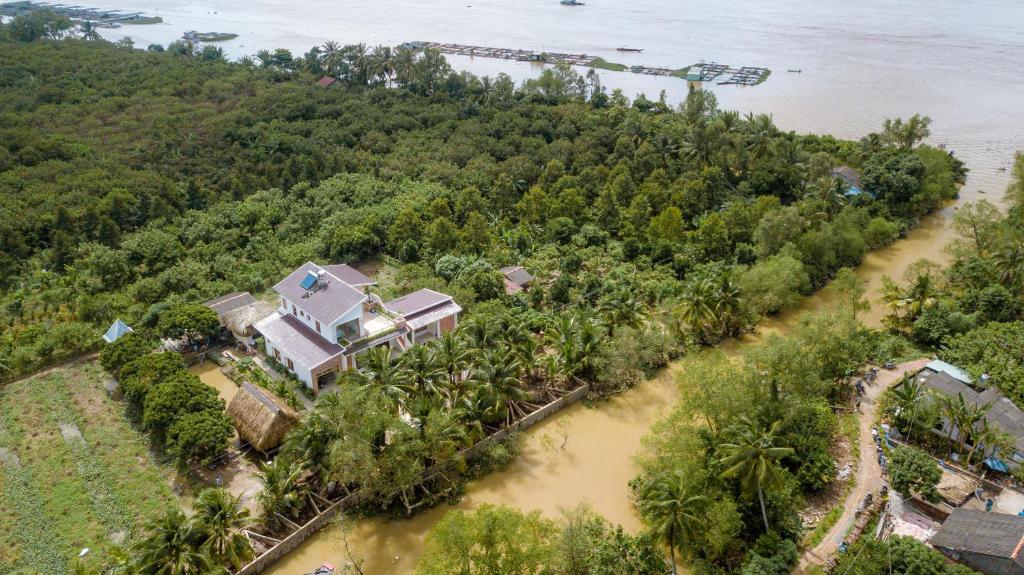This aerial photograph, likely taken from a drone, showcases a lush tropical landscape centered around a two-story white house with brown accents and a gray roof. The house is surrounded by dense greenery and features a thatch-roofed hut within its grounds. To the front of the house, a muddy waterway flows through, suggesting either a natural creek or possible flooding. Across this waterway, to the left, is a one-story house, while a field or large garden extends nearby. A circular driveway can be seen at the bottom right. The background reveals a vast body of water, presumably an ocean, with an inlet or dock area visible near the tree line. The entire scene is enveloped by a dense jungle, filled with palm trees and various bushes, extending from the front waterway all the way to the expansive ocean in the distance.